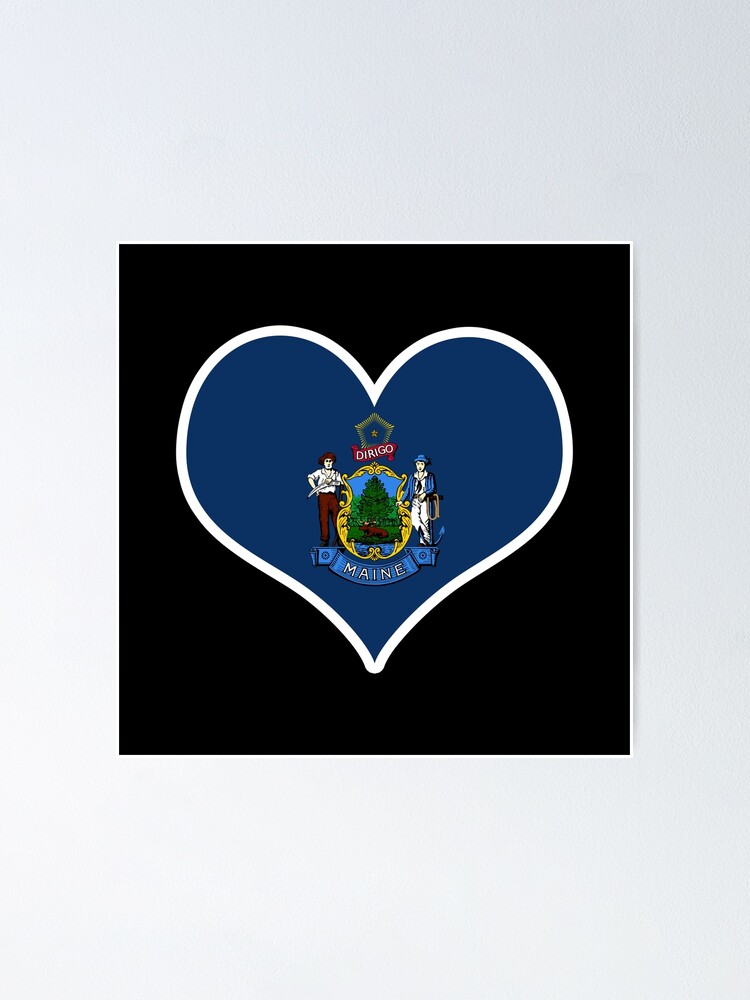This portrait-oriented image features a piece of artwork set against a light gray background. At the focal point, there is a centrally placed black square with a thin white border, housing a navy blue heart that also has a thicker white border. Inside this heart, a detailed insignia, which appears to be associated with the state of Maine, is displayed. The insignia includes two figures flanking an oval-shaped emblem; the left figure wears maroon pants and holds a large blade, while the right figure is dressed in a blue jacket. The emblem itself showcases a large pine tree with a brown animal, possibly a moose or dog, at its base. Above this scene, a hexagon-shaped design displays a yellow star with the word "DIRIGO" inscribed in white letters. Below, a blue banner reads "Maine" in white letters.